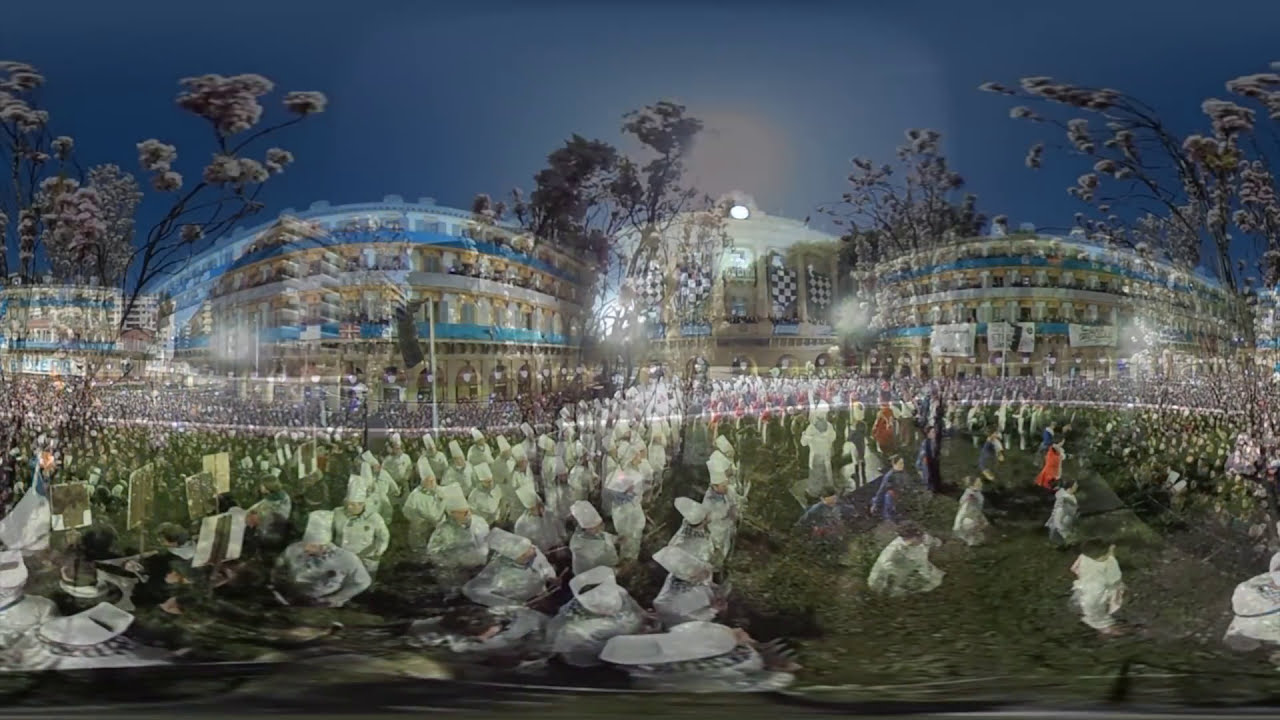In this heavily edited outdoor image, a surreal scene unfolds on a large green grass field dotted with trees budding with flowers. Hundreds of transparent chefs, clad in iconic white coats and tall hats, populate the area, giving the sense of a ghostly culinary gathering. In the backdrop, a massive, ethereal building resembling the Roman Coliseum with a mix of ancient and palace-like architecture stretches across the scene. This structure, characterized by blue accents and numerous windows styled with black and white checkerboard patterns, heightens the dreamlike quality of the image. Interspersed among the surreal elements are large, almost translucent flowers, enhancing the fantastical atmosphere. Overhead, a sky tinged with a purplish-blue hue, possibly hinting at sunset, completes this otherworldly tableau. The entire image seems like a fusion of multiple overlapping photographs, creating a disjointed yet captivating panorama.